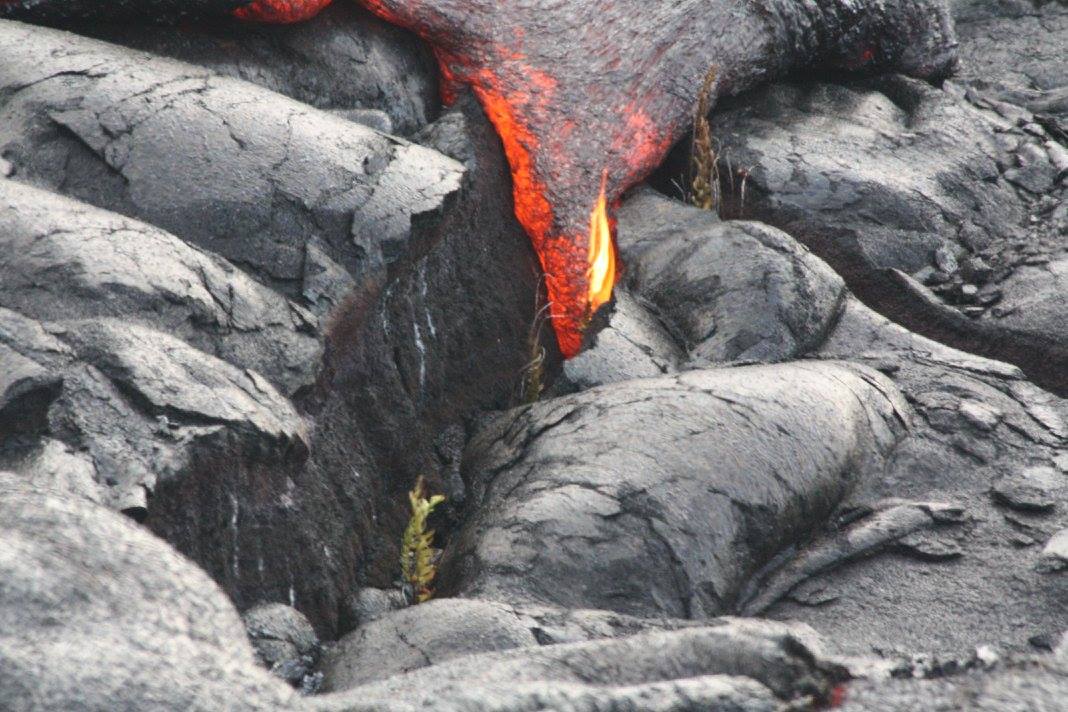This grainy, close-up photograph captures a dramatic and unique volcanic landscape, resembling a monochrome black and white image due to the predominant black and gray hues of hardened magma. The texture of the scene is matte with a hilly appearance riddled with cracks, suggesting a desolate, hostile environment. At the top middle of the photo, a vivid, red-hot lava is seen dripping and flowing, creating molten trails over the dark surface. This bright red and orange lava, almost like a tar-like substance, stands out strikingly against the charcoal background, with a small flame bursting from it in the center of the image. The lower middle to the right reveals tiny, fragile stalks of green foliage, struggling to survive before being inevitably consumed by the advancing lava flow. This juxtaposition of persistent life against the overwhelming force of the lava highlights the fierce and unyielding power of nature.